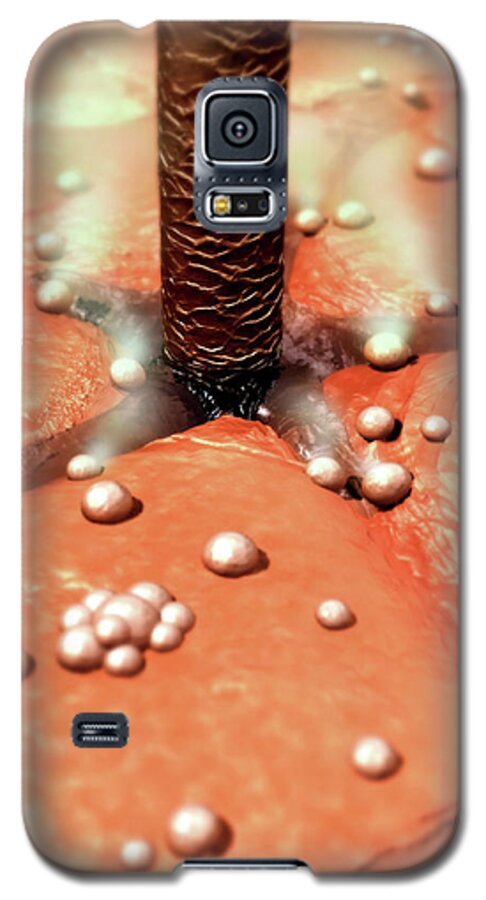This image is of the back of a Samsung Galaxy phone case with a unique and somewhat unsettling design. The case is primarily in cream, orange, and brown colors, resembling an orange creamsicle. The design prominently features a detailed, textured depiction that is subject to various interpretations. In the center, there is a crisscross pattern on what appears to be reddish, flesh-like skin, adorned with small, bulbous, pearl-like growths or droplets. Rising from this skin is a brown, textured element that resembles either a tree trunk, a bird's leg, or a hair follicle viewed under a microscope. This design extends near the camera lens and flash, adding to its unusual appearance. At the bottom, there is a cut-out section for the phone speaker. Overall, the distinctive case stands out, though its unsettling imagery might not appeal to everyone.